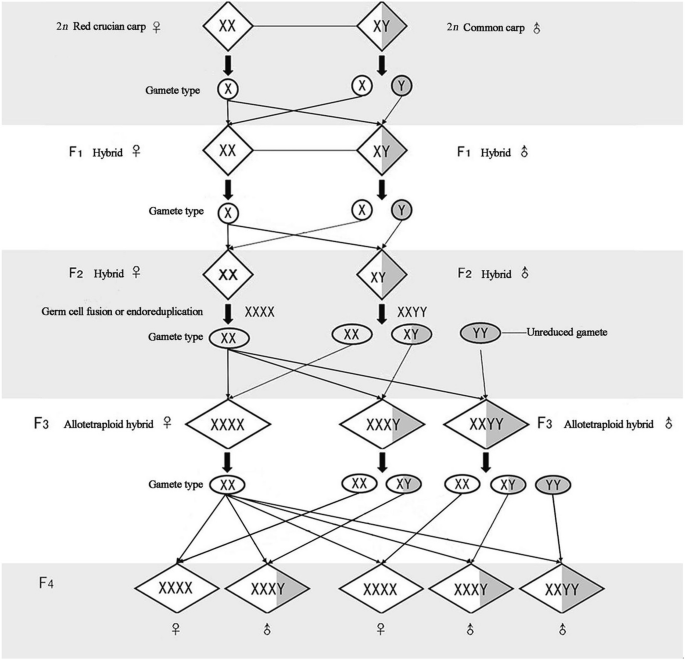The black and white diagram illustrates the various genetic combinations that can result from the mating of a red crucian carp and a common carp, focusing on their gamete types and hybrids. The background features alternating stripes of light gray and white, adding contrast to the detailed flowchart. At the top, the chart introduces two types of gametes: "2 Red Crucian Carp" on the left, represented by the XX chromosome, and "2N Common Carp" on the right, represented by the XY chromosome. Black arrows guide the viewer through the process, showing how the exchange of gametes can produce different hybrid combinations: XX and XY.

The left side of the chart contains diamond-shaped symbols for the red crucian carp, all in white, denoting the X chromosomes. On the right side, the common carp's diamonds are split between white and gray, representing the X and Y chromosomes respectively. If the common carp gives up an X chromosome, it results in an XX hybrid. Conversely, donating a Y chromosome results in an XY hybrid, which is male. Below this, the diagram explores further genetic processes such as germ cell fusion and endoduplication, leading to allotentraploid hybrids and additional gamete types. The chart eventually outlines five distinct combinations of male and female hybrids at the bottom, showcasing the variety of possible outcomes from this intricate genetic interplay.